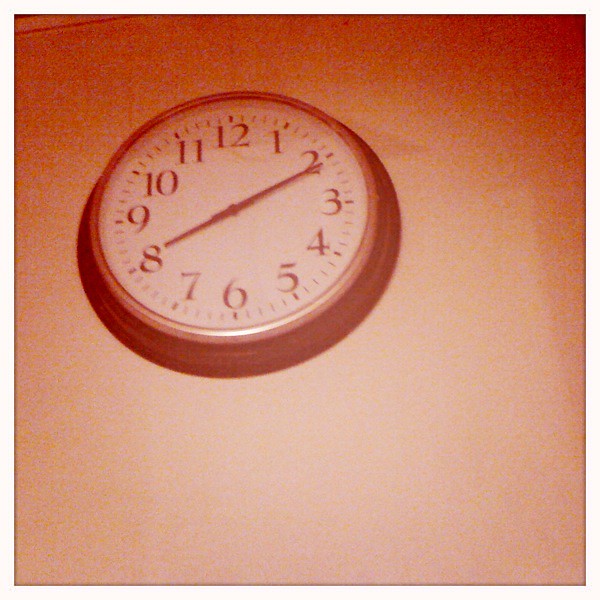This grainy, low-quality, square photo is meant to evoke a vintage, early Instagram aesthetic, complete with a sepia-toned filter resembling a Polaroid. The focal point is a simple, circular wall clock that you might find in a classroom. It has a black frame with a white face, black numerical markings, and black hands indicating the time is 8:11. The photo is taken from a low angle, looking up at the clock, and the top part of the clock's frame is not visible in the shot. The surrounding wall transitions from a deep orange at the top to a lighter orange and beige towards the bottom, creating a warm, nostalgic gradient effect. This gives the entire image a rust sepia tone and emphasizes the timeless, static nature of the clock against the softly tinted background.